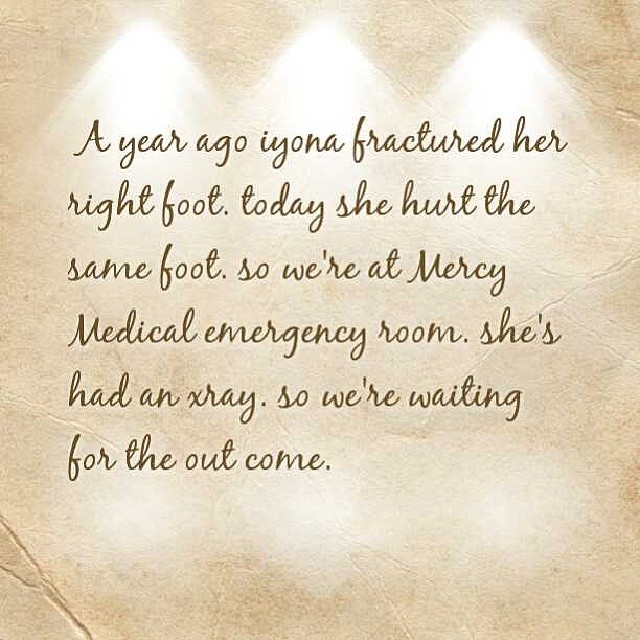The image features a computer-generated graphic designed to resemble a yellowed piece of paper with a stone-like background. It includes a cursive script in a darker brown color. At the top of the image are three white triangles, resembling emanating light. The background has subtle dark lines, adding a textured, stone-wall effect. 

The text reads: “A year ago, Iona fractured her right foot. Today, she hurt the same foot. So, we’re at Mercy Medical Emergency Room. She’s had an x-ray, so we’re waiting for the outcome.” 

The text appears as a statement likely intended for a social media post, providing a detailed update on Iona's medical condition.